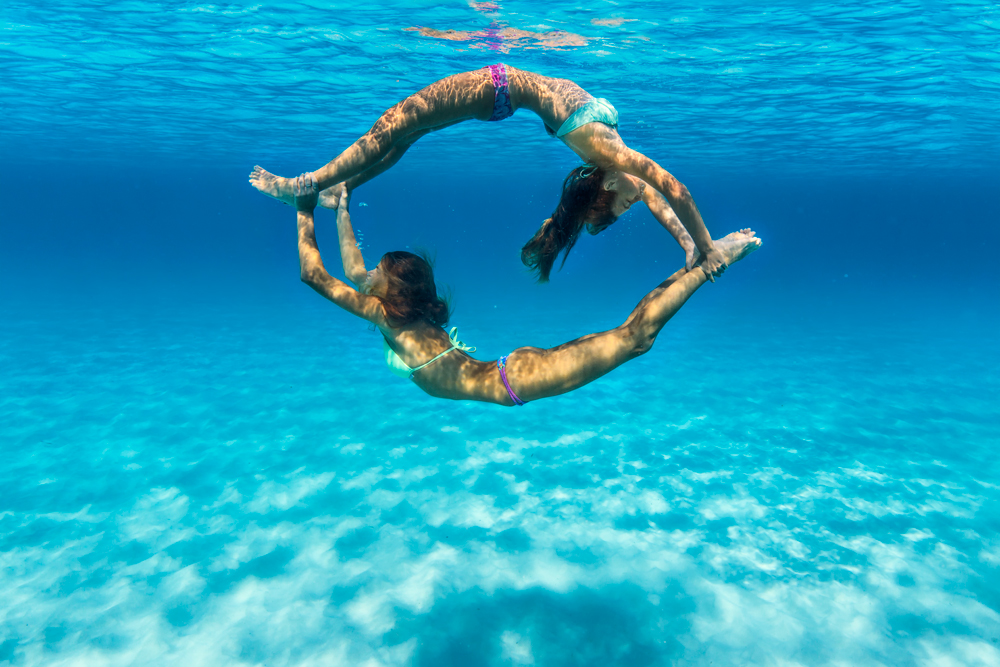In this underwater photograph, two teenage girls are performing an acrobatic trick in crystal-clear blue water. They are grasping each other's ankles, creating a circular "O" shape with their arched bodies; one girl's stomach faces the water's surface while the other's faces the pool floor. Dressed in light blue or teal bikini tops and purple bikini bottoms, the girls' dark brown hair contrasts; one has hair tied in a bun and the other in a ponytail. Ripples and sunlight play on the water's surface above them, while bubbles rise from their exhalations, adding to the dynamic, lively scene. The clarity of the water obscures any pool edges, making the setting seem vast and open.